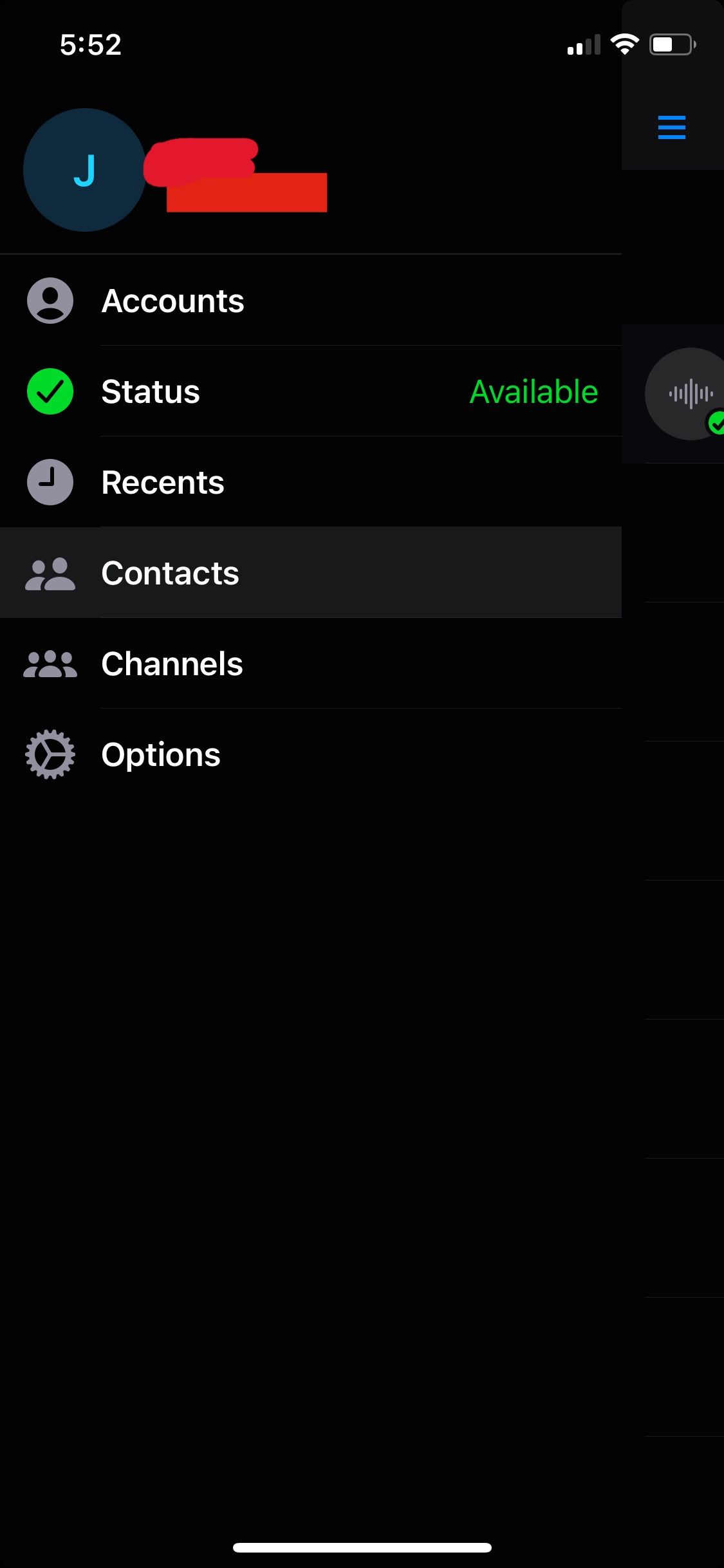This is a detailed and cleaned-up descriptive caption for the provided image:

"In the screenshot taken from an iPhone, which appears to be of a social media app similar to WhatsApp, the background is predominantly black. At the top left, the time is displayed as 5:52, while the top right corner shows the cell phone signal icon, Wi-Fi icon, and battery icon. 

The main app interface shows a display picture icon with the letter 'J' in bluish text against a dark blue background, though the user's name has been obscured with red scribbles. To the far right of the display picture is a drop-down menu icon.

Below the display picture are several menu options arranged in a line:
1. **Accounts**
2. **Status** - This option has a green checkmark and text indicating "available" in green.
3. **Recents**
4. **Contacts** - Surrounded by a light gray bar, suggesting it is currently selected.
5. **Channels**
6. **Options**

The rest of the screen below these options is empty."